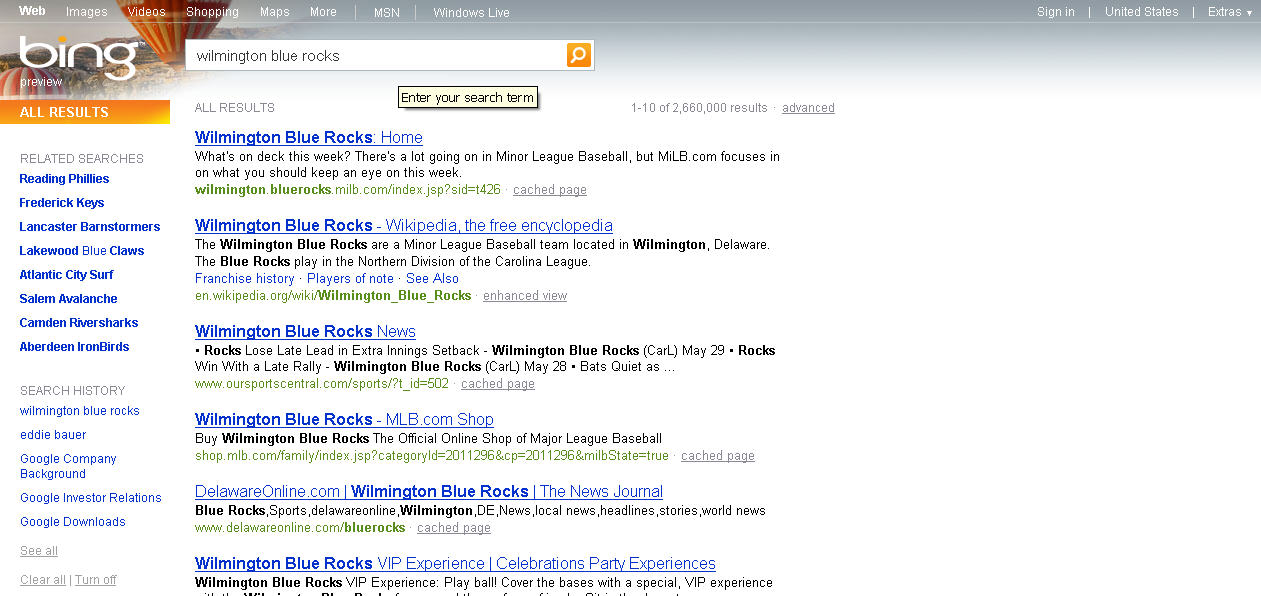This image is a screenshot taken from the Bing search engine page in preview mode. The Bing logo is displayed in lowercase letters with an orange dot above the "i" while the rest of the text is in white. At the top of the page, there are navigation tabs labeled "web," "images," "videos," "shopping," "maps," "more," and additional links to "MSN" and "Windows Live." The top-right corner includes options for "sign in," "United States," and "extras."

The search query at the top, "Wilmington Blue Rocks," is displayed within the Bing search bar under the prompt "enter your search term." The search results consist of blue clickable links with green URLs beneath them. The first search result header reads "What's on deck this week?," and the description mentions updates and highlights for minor league baseball, specifically focusing on MILB.com, which offers insights into notable events and happenings throughout the week. The page continues with more search results relevant to the Wilmington Blue Rocks.